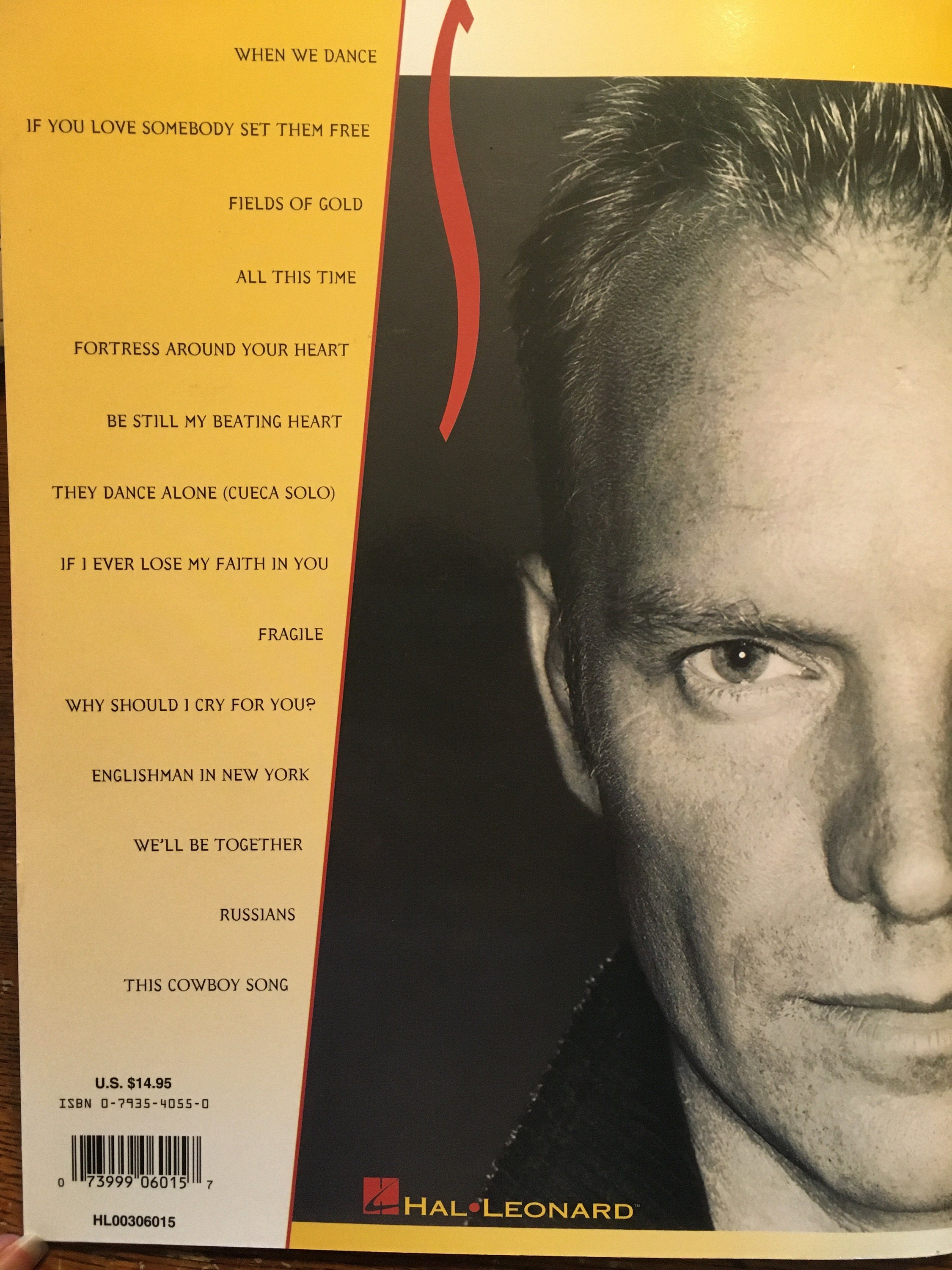The back cover of the album is a vertical rectangle featuring a color palette of yellow, beige, and red. Dominating the right side of the cover is a black-and-white photograph of a man with short, highlighted hair, presenting an intense, forward stare and showing only half of his face, from his hairline to his chin. Along the left side, in black text, is a list of song titles which includes "When We Dance," "Fields of Gold," "All This Time," "If You Love Somebody Set Them Free," "Fortress Around Your Heart," "Be Still My Beating Heart," "They Dance Alone (Cueca Solo)," "If I Ever Lose My Faith in You," "Fragile," "Why Should I Cry for You?," "Englishman in New York," "We'll Be Together," "Russians," and "This Cowboy Song." The name 'Hal Leonard' appears at the bottom, presumably indicating the producer of the album. Additional elements, such as price information, the ISBN number, and a barcode, are located in the bottom right corner. Notably, there is also a large red "S" just to the left of the man's photograph.